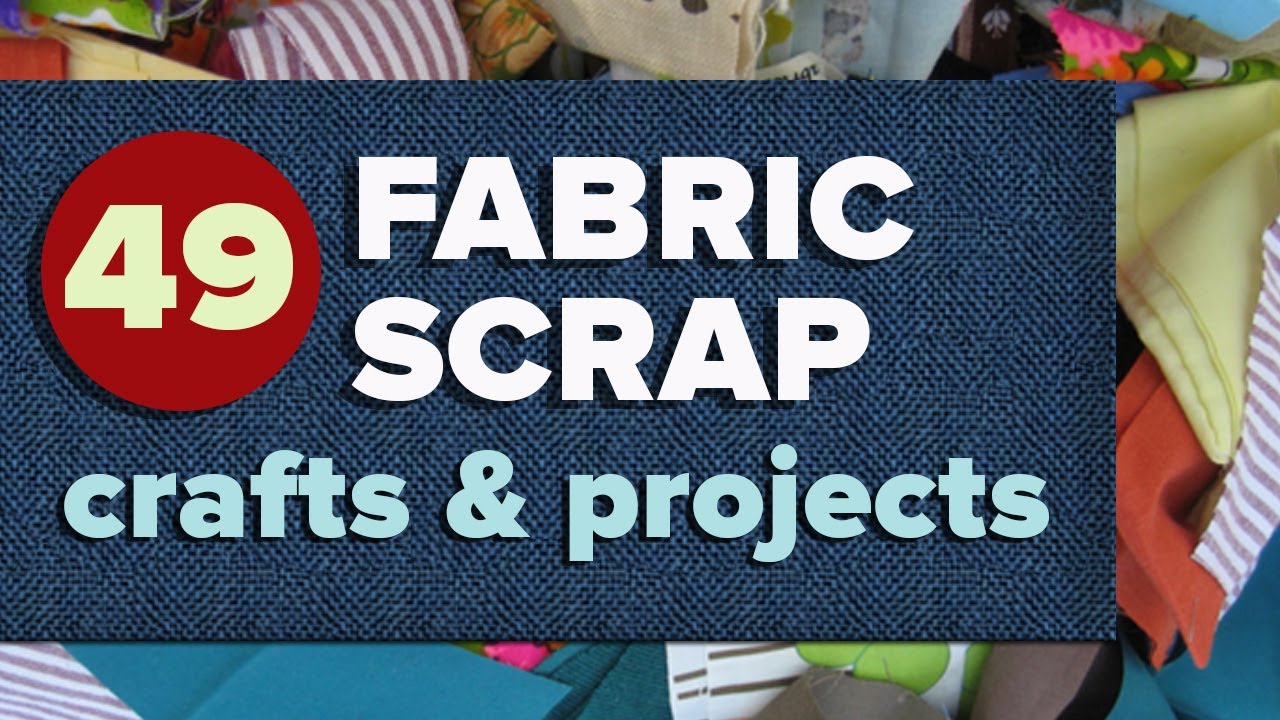The image depicts the title page of an artist's craft book featuring a vibrant collage of various fabric scraps. The background showcases an assortment of colorful textiles, including striped pink and white, light yellow, dark orange, brown and white, teal blue, cream-colored with brown polka dots, and floral patterns with pinks and greens. Centrally placed is a blue woven rectangular fabric patch, taking up about 75% of the image, aligned slightly to the left. Within this patch, the book title "Fabric Scrap, Crafts and Projects" is stylized with 'Fabric Scrap' in white font, and 'Crafts and Projects' in light blue. A red circle containing the number '49' in a light yellow font overlays this patch, adding a distinct focal point. The intricate design and layered fabrics capture the essence of the craft projects detailed within the book.